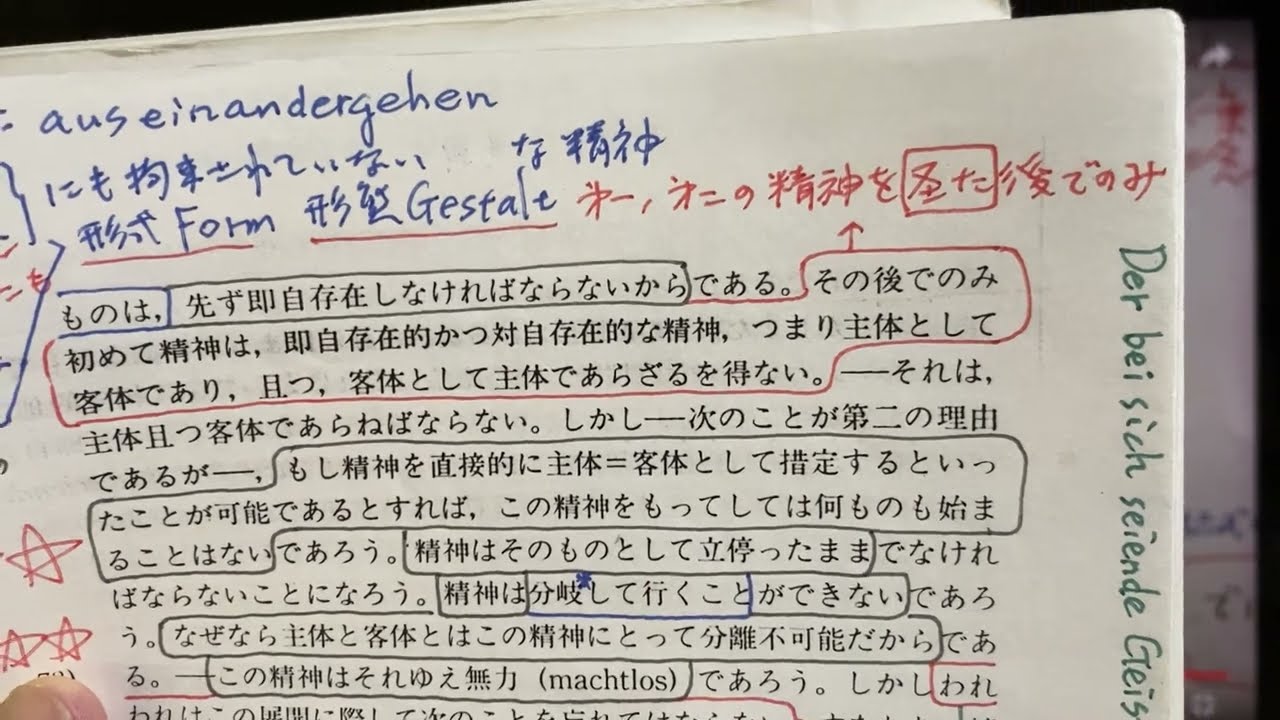This image portrays a zoomed-in view of a document, seemingly a homework sheet, held up by someone's thumb visible in the bottom left corner. The paper itself features a striking mix of printed and handwritten text in various fonts and inks. At the top, in blue ink, the document displays the word "AUSEINANDERGEHEN." Below this, one line of Asian characters is followed by another line with additional Asian characters. To the right of this third line, there are handwritten Asian characters written in vivid red ink. Scattered among the numerous lines of black text are characters circled in both black and red ink, while to the left of these characters some are marked by red stars. On the very right side of the page, the letters "DERBEISICHSEIENDEGEIS" run vertically in ink. Additionally, in the blue handwriting on the page, the words "FORM" and "GESTALT" are readable, hinting at possibly multilingual notes, potentially from a German-speaking student learning an Asian language, such as Chinese or Japanese.